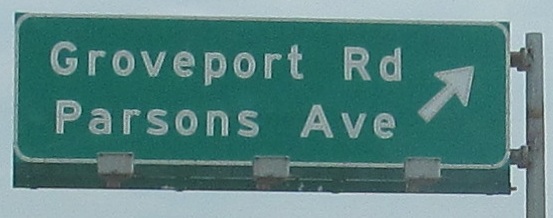The image features a rectangular street sign, prominently displayed with directional information. The sign has a green background with a white border and is affixed to a pole on the right side. The top line of the sign reads "Groveport Road RD" in bold white letters, and directly below it, "Parsons Avenue AVE" is written in the same white font. Additionally, a white arrow on the sign points upward and slightly to the right, indicating the direction. The sign is securely fastened with three brackets along the bottom edge, ensuring stability.